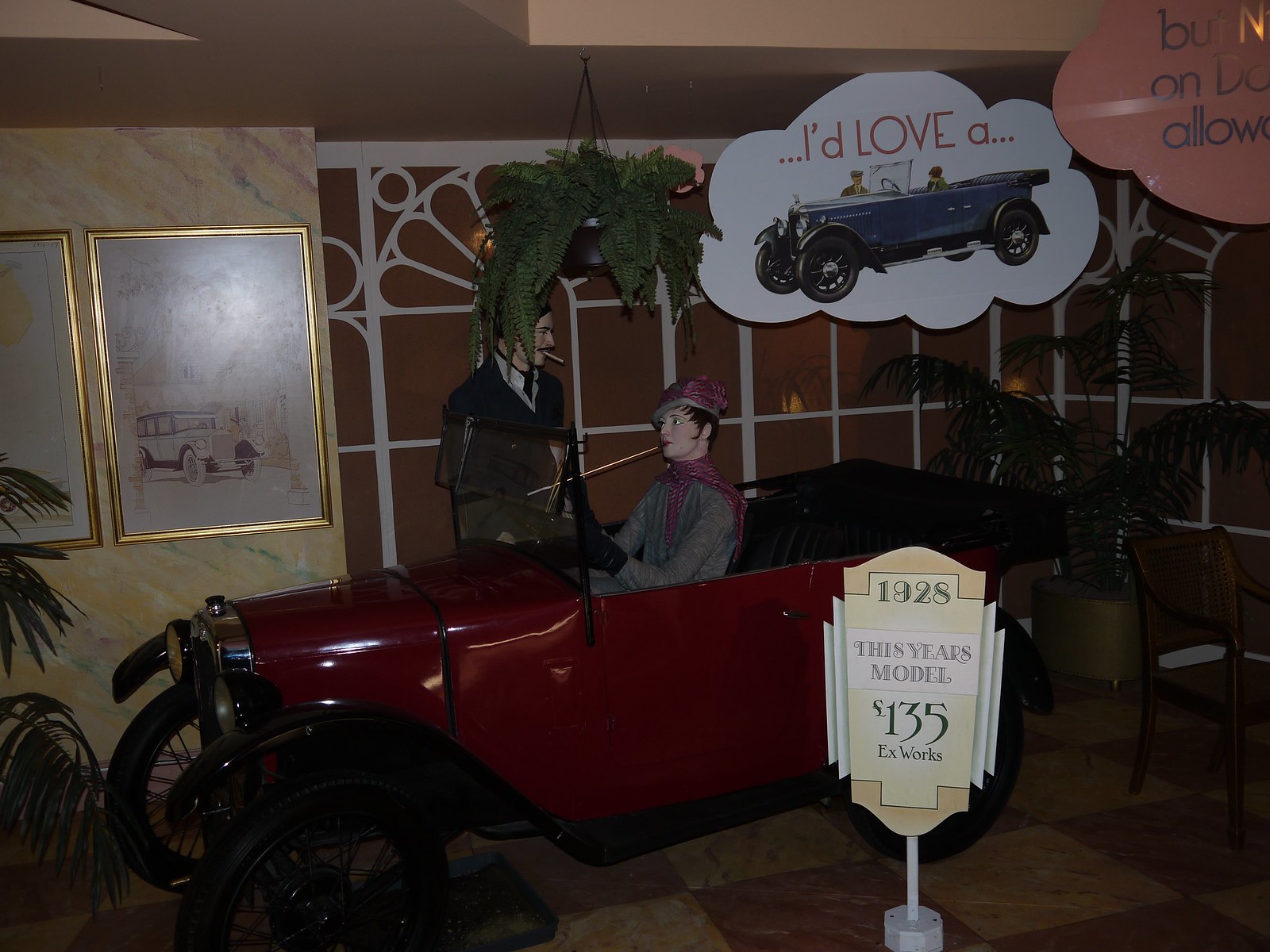This image captures a detailed indoor museum exhibit showcasing a 1928 red Model T car. The main focus is on the vintage vehicle, which is marked with a sign reading "1928, This Year's Model, $135." The display features two mannequins: a woman seated in the driver's seat and a man standing beside her. The woman, dressed in period attire, appears to be holding or smoking a vintage cigarette. The man, also clad in era-appropriate clothing, gazes at her with a cigarette in his mouth. Behind them is a red backdrop meant to resemble a decorative fence, adorned with bubble plaques. One plaque reads “I’d love a” accompanied by an image of another antique car. The scene is accented by a wall on the left displaying pictures of other old cars, creating an immersive presentation of automotive history from the 1920s.